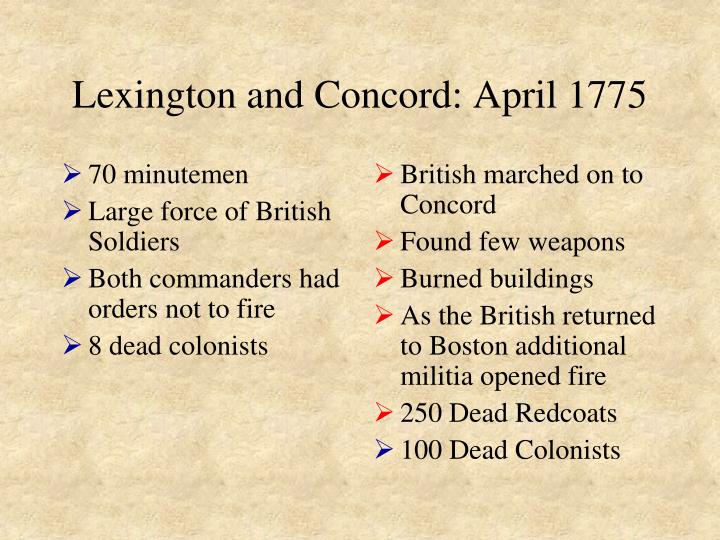This image depicts a detailed infographic, seemingly from a Microsoft PowerPoint presentation, designed with an aged parchment-like digital background. The text, centered on this tan backdrop, provides a chronological account of the events at Lexington and Concord in April 1775, an early and significant episode in the Revolutionary War. At the top, in a thin black font, the title reads: "Lexington and Concord, April 1775."

On the left side, blue arrows precede each bullet point: 
  - 70 Minutemen
  - Large force of British soldiers
  - Both commanders had orders not to fire
  - Eight dead colonists  

On the right side, red arrows accompany the text: 
  - British marched on to Concord
  - Found few weapons
  - Burned buildings  

Further down, describing the aftermath as the British returned to Boston:
  - Additional militia opened fire
  - 250 dead redcoats 

A final point, marked by a blue arrow:
  - 100 dead colonists 

This infographic effectively summarizes the pivotal skirmishes and their tragic consequences, laying out the narrative with a clear and historical focus.